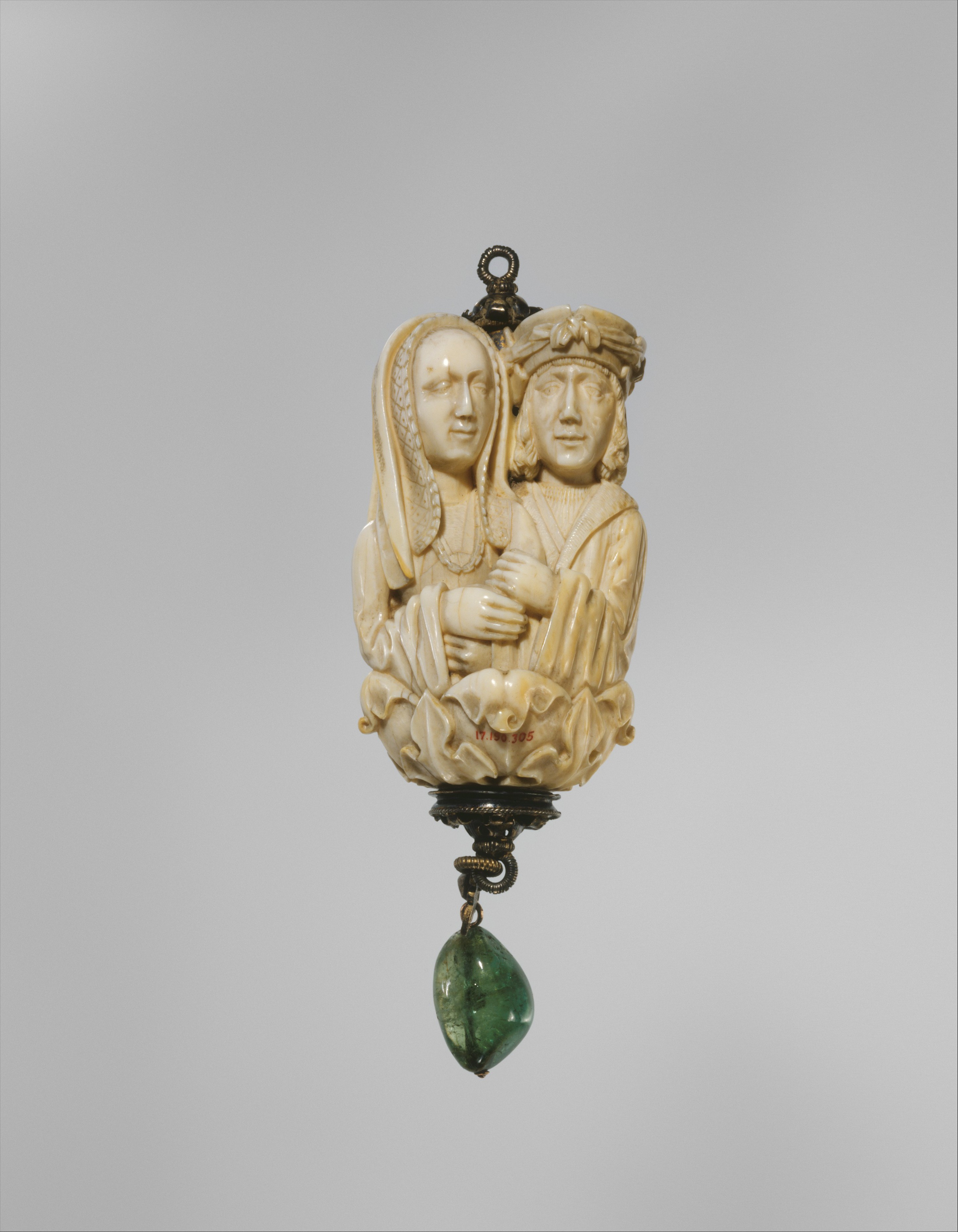The image shows a meticulously handcrafted figurine, likely intended for decorative or religious use, with a gray background. The centerpiece is an ivory or beige marble-like carving of two individuals from ancient times, perhaps reminiscent of Shakespearean characters. The figure on the left appears to have long hair covered by a scarf, while the figure on the right wears a distinctive hat with a ribbon, often described as a turban. Both are depicted holding hands and sitting atop a large, intricately carved white marble rose. Below this scene is a dark metal extension with a small chain, ending in a dark green stone or blue glass pendant. At the top of the figurine, there is a small hook, suggesting it can be hung as a piece of wall art, part of a lamp, or a large pendant necklace. The craftsmanship of this piece is notably exquisite, reminiscent of detailed handiwork often seen in religious artifacts.